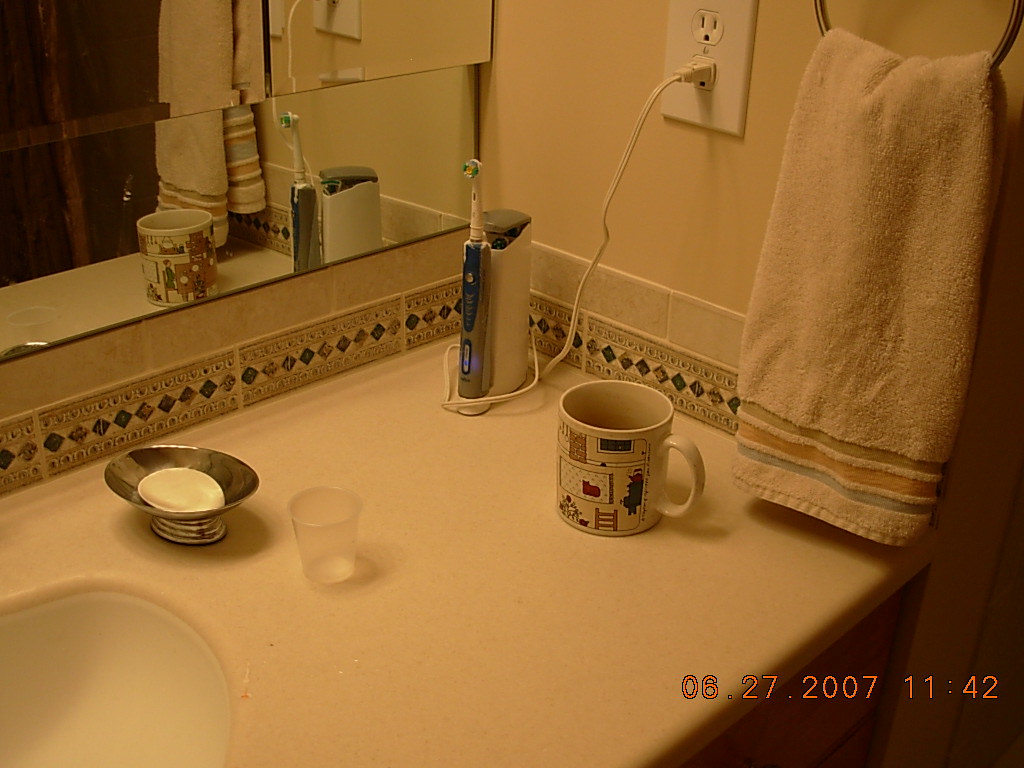This indoor color photograph captures a detailed view of a bathroom sink and countertop from a corner perspective. The white countertop extends towards the lower left, where a portion of the sink is visible. Prominently positioned in the upper right corner, slightly off-center, is an electric toothbrush nestled in its holder, with its power cord wrapped around and extending diagonally to an American wall outlet located just right of center.

In the far upper right, part of a towel hoop is visible, holding a neatly folded towel featuring three horizontal stripes. Nearby, approximately center image and to the left of the towel, stands a ceramic coffee mug decorated with a pattern, appearing empty.

A mirror spans from the left center background to the upper left edge, reflecting the central and right-hand items. The mirror comprises two thin, rectangular pieces of glass, deliberately separated—not cracked—adding a unique visual element.

In the lower left quadrant, close to the sink's edge, a silver soap dish holds a white bar of soap. Adjacent to the soap dish, to its right, sits a small clear plastic cup, likely three or four ounces in size.

An orange timestamp overlay is present, indicating "06.27.2007 11:42," providing both a date and time for the photograph.